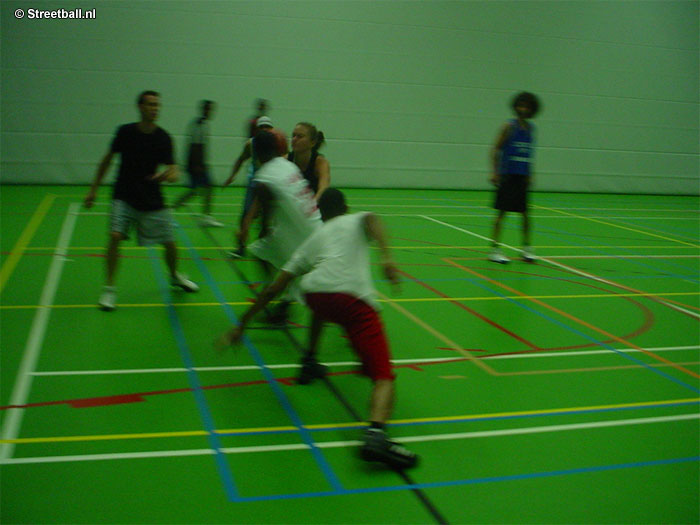The photo depicts an indoor sports gym with a green cinder block wall and a vibrant green court marked with a variety of lines in different colors, including yellow, green, orange, blue, and red, suggesting multiple sports could be played there. In the upper left corner, there is white text reading "copyright streetball.nl." The scene is slightly blurry, adding a sense of dynamic motion. Nine individuals are present: three in the foreground and six in the background. A man with black shoes and red shorts lunges to the left with an outstretched arm, attempting to take a basketball from another man in a white short-sleeved t-shirt. Near them, a blonde woman appears to be defending. Additional lines and shapes on the court, such as rectangles and semi-circles, add to the complexity of the setting. In the background, a mix of men and women dressed in athletic wear, some possibly engaged in the action, are partially visible. The composition hints at an intense and energetic sporting moment inside a versatile gym space.